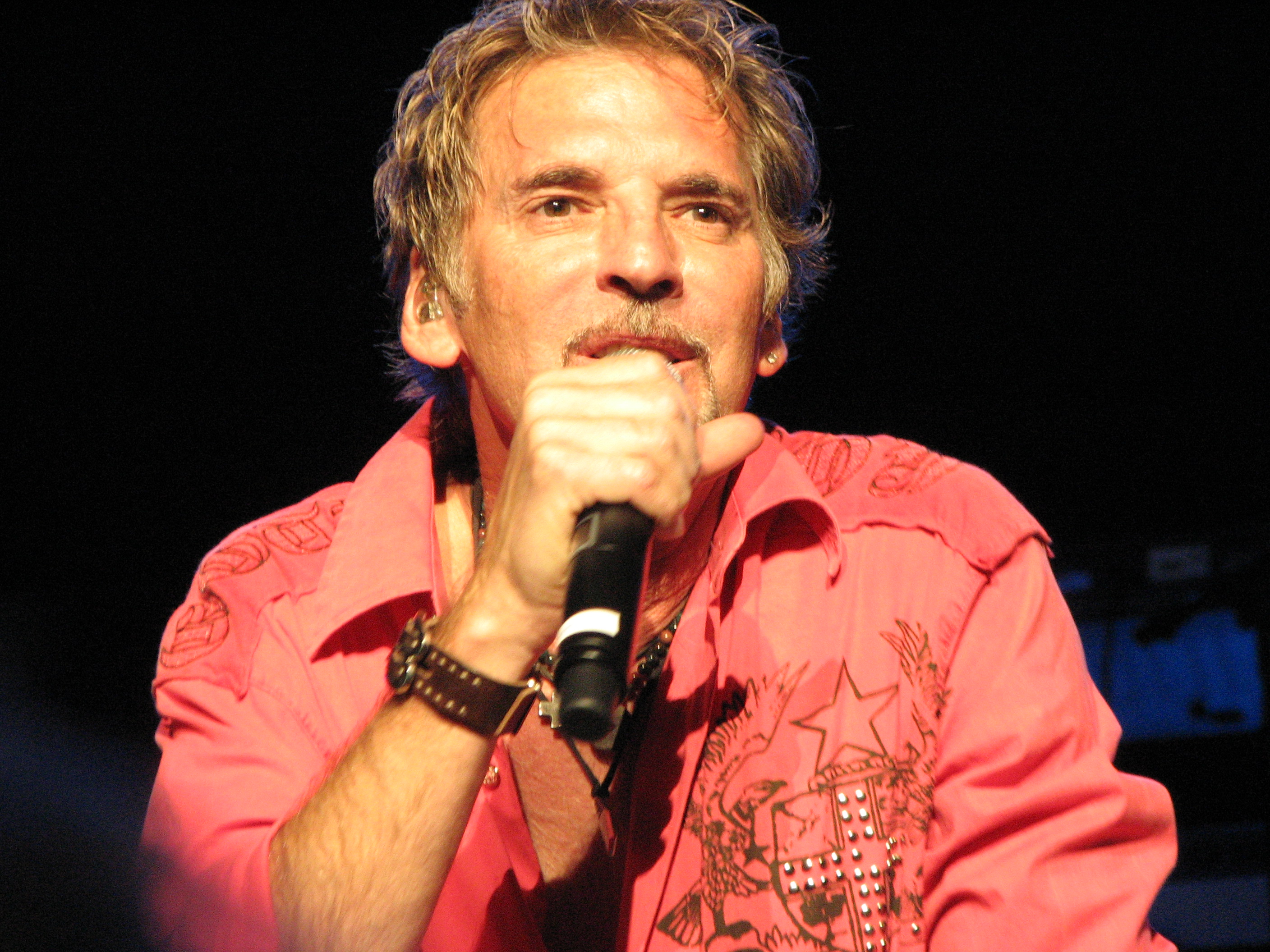In the image, a man with sandy grayish-blonde, medium-length hair and a brownish-blonde mustache, along with sideburns, is depicted holding a microphone close to his mouth as he either sings or speaks. He appears to be wearing a pinkish-reddish, salmon-colored western-style shirt with a collar and long sleeves that have been casually rolled up. The shirt is unbuttoned low, revealing some chest hair. On the left side of his chest, there's a prominent star with what seems to be bedazzled or sequined decorations, possibly forming a cross with beadwork. 

The man also sports several necklaces and a leather watch on his right wrist, characterized by holes on both sides. Visible in his ears are in-ear monitors, suggestive of a stage performance. His facial expression is intense, possibly indicating a passionate moment in his performance. The backdrop is dark, predominantly black with a swatch of blue, emphasizing the stage-like atmosphere.